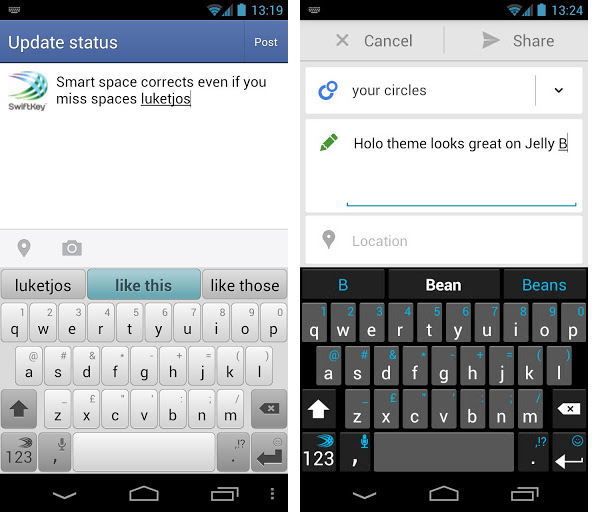This side-by-side image comparison showcases two different smartphone screen displays. The left screen features a user interface designed for updating status or posting, as indicated by a blue banner just below a black header. The main background is white, prominently displaying a backward C-shaped logo with intertwined blue and green lines, symbolizing the SwiftKey app. To the right of this logo, text reads "SwiftKey" followed by a description, "Smart Space corrects even if you miss spaces," accompanied by a misspelled word as an example. The bottom section of this screen captures an image of a keyboard interface.

The right screen presents a different interface. It has a gray top border with "Cancel" and "Share" options flanking enclosures reminiscent of action buttons. Beneath this gray header lies a white rectangular region displaying two overlapping blue circles—one large and one small, positioned diagonally. Beside these circles, the label "Your Circles" is visible. This is followed by another white rectangular section featuring a green pencil icon diagonally oriented towards the upper right corner, with text next to it proclaiming, "Holo theme looks great on Jelly Bee." The lower portion of this screen similarly shows an image of a keyboard, but this time with a black background and gray keys, differing from the left screen's keyboard appearance.